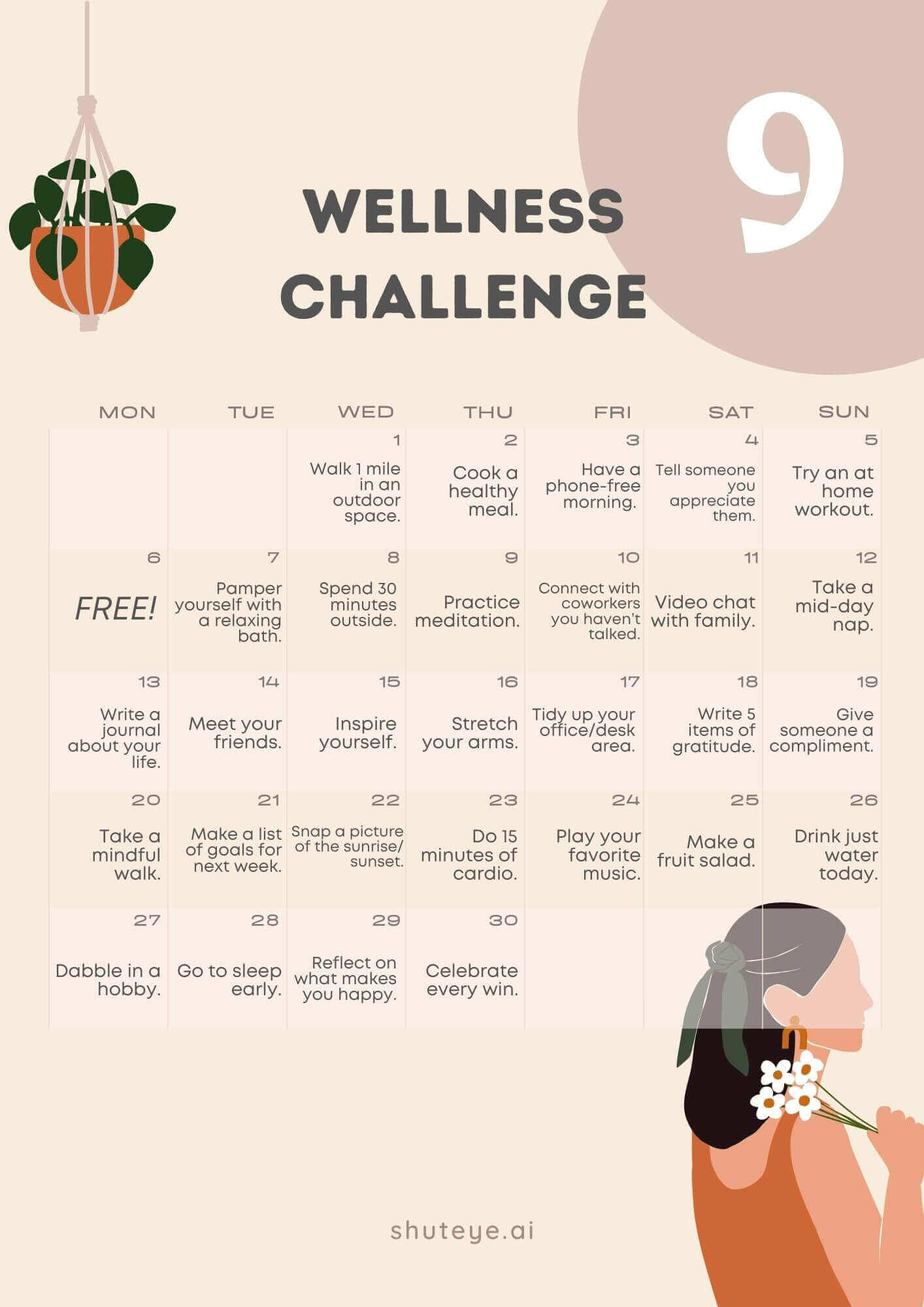The image is a detailed calendar designed to promote wellness activities. At the top left, there's a charm hanging from a rope. Below this charm, there is a plant in an orange pot with dark green leaves. The rope above the plant is light brown. 

To the right, the word "Wellness" appears in light black text. At the top right corner of the image, there is a circular shape resembling a sun, colored in a pinkish-salmon hue, with the number "9" displayed in white.

The center of the image features the actual calendar, which covers from Monday to Sunday and includes various wellness activities. Each day has dedicated activities written in small squared boxes. For example, Wednesday the 1st instructs to "Walk one mile", the 2nd suggests "Cook a healthy meal", followed by "Have a phone-free morning", "Tell someone you appreciate them", and "Try an at-home workout". Subsequent days prompt activities like "Pamper yourself", "Spend 30 minutes outside", "Practice meditation", "Connect with coworkers", "Video chat", and "Take a midday nap", continuing through to the 30th of the month.

Additionally, there is an image of a woman holding flowers located at the bottom right of the calendar.